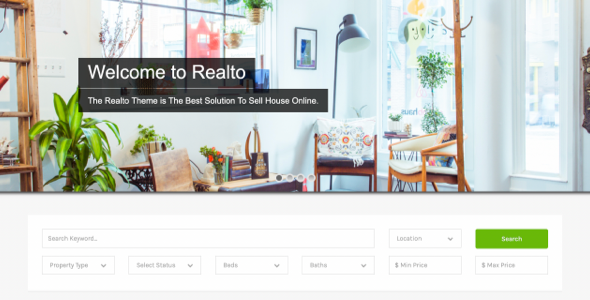The image depicts a room with a light blue-colored wall as its backdrop. In the scene, a wooden ladder leans against the wall, adding a rustic touch to the decor. There's a window adorned with several flowerpots, some hanging and others sitting on the ledge, introducing a hint of greenery. The room also features a couple of chairs and a striking, large black lamp with a long, slender stand elevating it off the ground. To the right of the window, additional windows let in natural light, and a coat rack stands nearby.

A black box with white text prominently displays the message, "Welcome to RealToe," indicating the RealToe theme, which is touted as the best solution for selling a house online. Beneath this message, the background turns gray, and a white box is present with various interactive elements. The top of this white box features a text box labeled "search keyword." Following this are drop-down menus labeled "property type," "status," and other options that are too blurry to decipher clearly, along with drop-down menus for "location," "minimum price," and "maximum price."